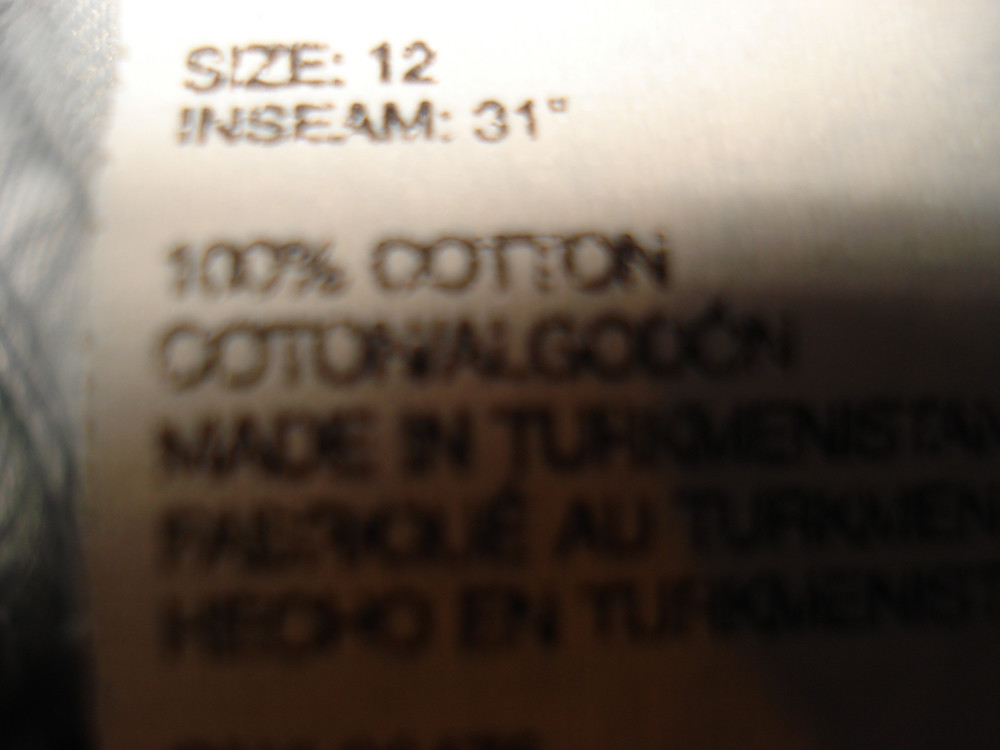A close-up image captures the intricate details of a clothing tag situated inside a garment. The white tag, adorned with black text, reveals its information clearly at the top, where the size is noted as 12, followed by an inseam measurement of 31. The lower portion of the tag, partially obscured by shadows, informs the viewer that the material is 100% cotton. The phrase "Made in" is faintly visible but obscured enough to make the country of origin indiscernible. The left edge of the tag has a texture that suggests it is attached to a pair of jeans, which is subtly confirmed by the appearance of denim fabric peeking into the frame. The shadowy gradient, growing darker from the center towards the bottom right, adds a touch of mystery to the image's overall aesthetic.